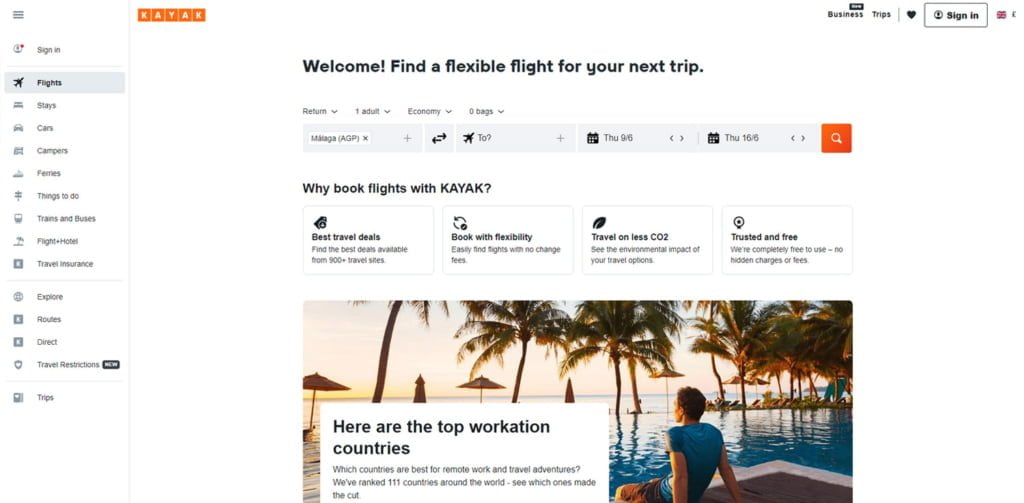Welcome to the flight booking section of a travel website that functions similarly to Kayak, featuring an interface dominated by an orange and white color scheme. Each letter in the website's name is encased in its own white box. On the left side, though not exactly in the corner, there's a menu icon comprising three stacked lines. Below this icon, the navigation bar includes options like "Sign In," "Flights," "Stays," "Cars," "Campers," "Things to Do," "Trains and Buses," "Flights and Hotels," "Travel Insurance," "Explore Routes," and "Direct Travel Restrictions."

The screen prominently displays a welcome message encouraging users to find a flexible flight for their next trip. The search interface is already partially filled out for a flight starting from AGP, with the specifics of one adult, economy class, and no checked bags. The destination field appears to be awaiting input, marked by a question mark. The dates listed are somewhat unclear, possibly indicating a range either from Thursday, 9/5 to 16/5, or 9/6 to 16/6.

An orange button labeled "Search" is positioned below the date range input fields, ready to initiate the search query. Following this, the site highlights reasons to book flights through their platform, emphasizing advantages such as the best travel deals, booking flexibility, reduced CO2 emissions, trustworthiness, and being free to use. The page concludes with a section titled "Top Workation Countries."